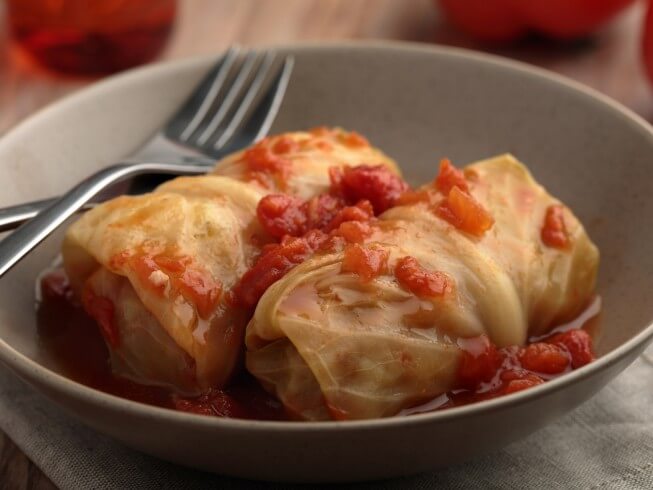This photorealistic image features a beautifully plated dish that could easily grace the pages of a gourmet magazine. Two cabbage-wrapped rolls, their translucent white leaves tenderly cooked, rest invitingly in a light gray bowl. These rolls, reminiscent of egg rolls in shape and appearance, are generously topped with a chunky, vibrant red tomato sauce. The tomatoes, either crushed or diced, are particularly concentrated in the middle of the wraps, adding a rich texture to the presentation. The bowl is adorned with a silver fork, positioned on the left side and partially obscuring another utensil, possibly a knife. The entire setting is laid out on a pristine white tablecloth, suggesting a sophisticated dining experience, possibly at a wedding or upscale restaurant. The background hints at additional table elements, like drinking glasses or a vase, enhancing the overall elegance of this culinary scene.